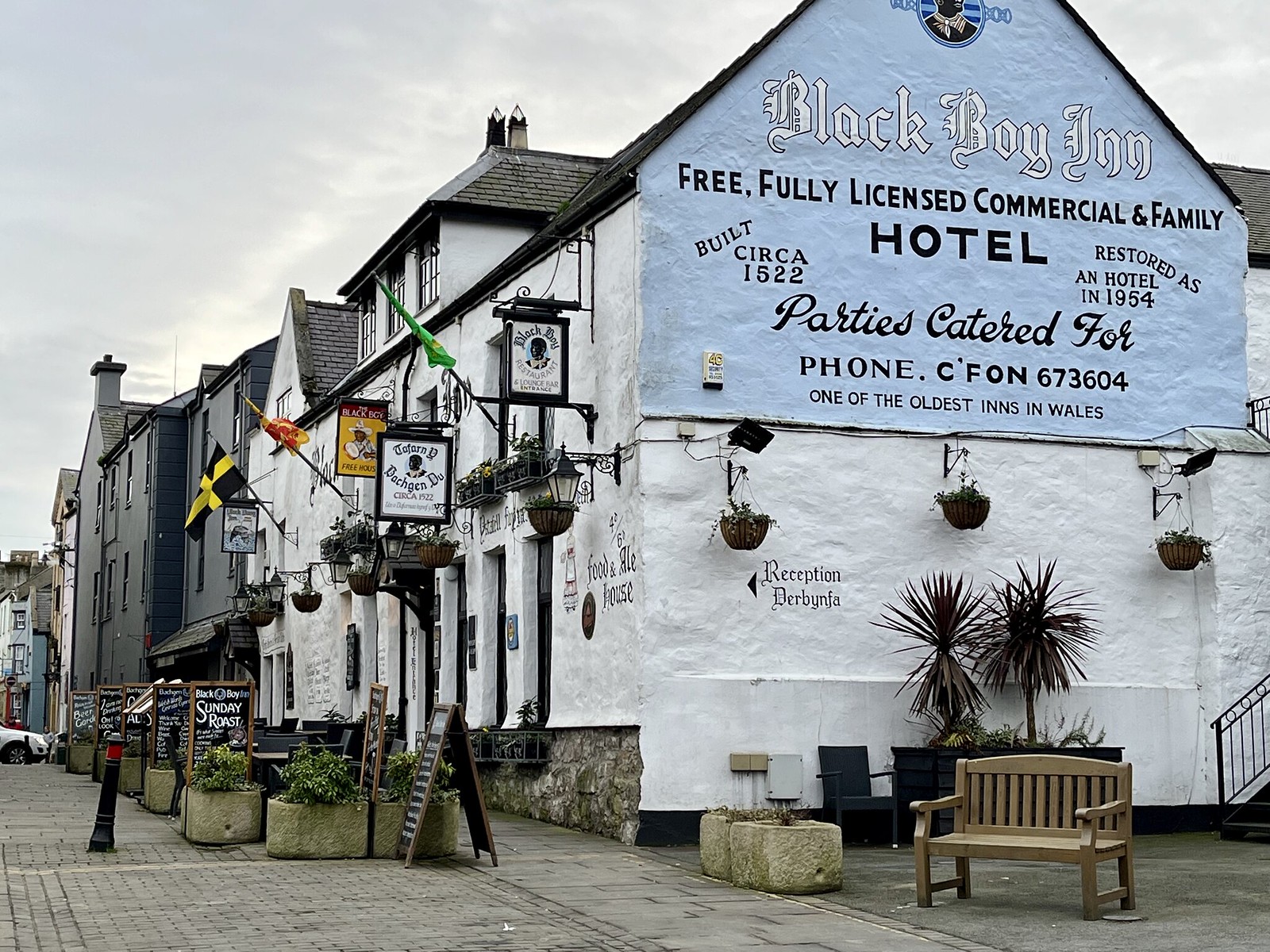The photograph depicts an old, multi-story building that has served different purposes over the centuries. The building, boasting white, rough-textured stone walls and a black-tiled triangular roof, is currently branded as the "Black Boy Inn." Prominently displayed on a light blue section of the upper wall is white text that reads, "Black Boy Inn, free fully licensed commercial and family hotel, built circa 1522, restored as a hotel in 1954, one of the oldest inns in Wales." Below these inscriptions are additional details, including "parties catered for" and a contact number, "CFON 673-604." The building's exterior is adorned with hanging baskets filled with flowers and flagpoles, one bearing a dark navy blue flag with a yellow cross. The surrounding area features cobblestone sidewalks, some outdoor benches, and signs indicating the presence of additional businesses, such as cafes, hinting at a vibrant community atmosphere.